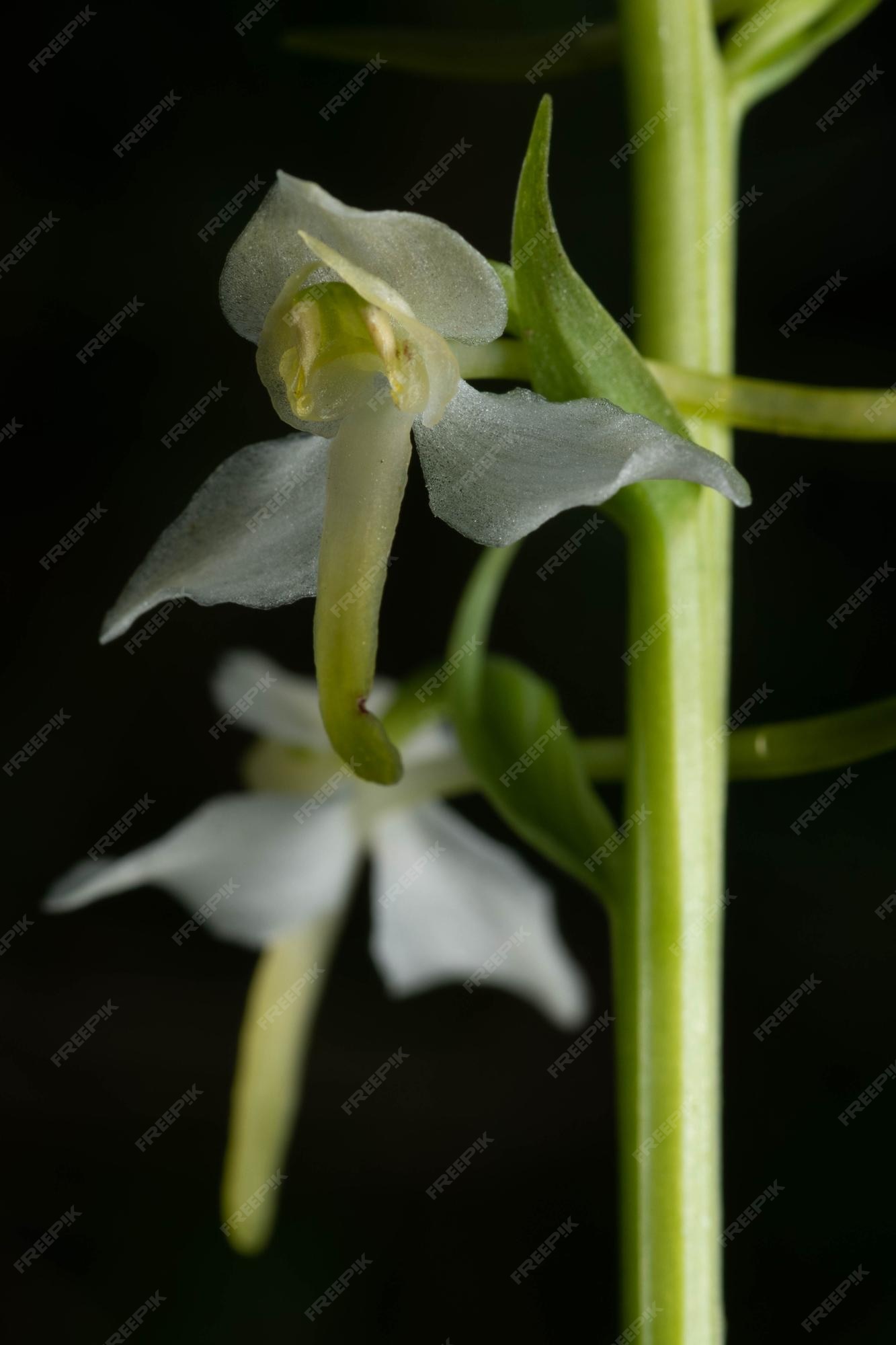This color photograph is a detailed close-up of two orchid blossoms against a stark black background. One flower is in sharp focus, while the other remains blurred in the background. Each blossom has three pristine white petals: one at the top and two on either side. Emerging from the center is a tongue-like structure that is pale green, transitioning to a darker shade at the tip. The flowers also feature small, pale green leaves near their bases, attached to a long, robust green stem. Overlaid diagonally across the image is a translucent gray watermark that reads "free pick."